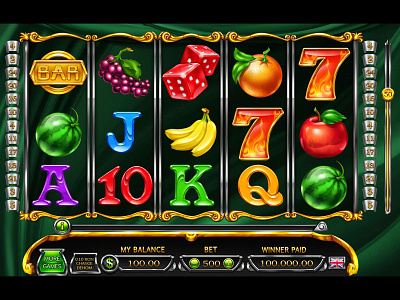This is a screenshot of a colorful fruit-themed slot machine game available for play on both computer and cell phone. The image features five columns of slots with distinct symbols and three rows, all framed by thin black borders on the top and bottom. Each column contains a variety of fruits and classic slot machine symbols. From left to right, the symbols include: a gold bar, a green watermelon, and a purple A; a bunch of grapes, a blue J, and a red 10; two red dice, a bunch of bananas, and a green K; an orange, a flaming red 7, and an orange Q; and another flaming red 7, a red apple, and a green watermelon.

Additionally, the left and right sides of the slot grid are adorned with little boxes containing different numbers, although the numbers aren't clearly discernible. The background features a greenish hue, enhancing the vivid colors of the symbols, while each column is topped with golden ornate squiggles.

At the bottom of the screen, a green pot icon is displayed, along with key game metrics: the player's balance stands at $100, the current bet is $500, and the winner paid amount is $100,000. A small British flag is visible, adding a touch of international flair. This detailed snapshot encapsulates the visual and functional elements of the slot machine game, although it appears that no winning combination has been achieved in this particular round.